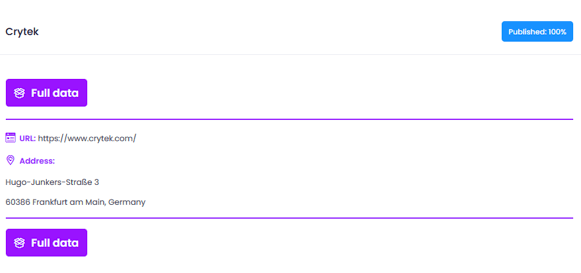This image is a screenshot of an informational screen. In the upper left-hand corner, the logo "Crytek" (C-R-Y-T-E-K) is displayed prominently. On the upper right-hand corner, there's a blue button indicating "Published 100%". Below it, a light gray line separates this section from the next.

On the following row, situated on the left, there's a prominent purple button labeled "Full Data", alongside a purple line running horizontally. Further down, the URL "https://www.crytek.com" is provided, accompanied by an icon suggestive of a website next to the URL. 

Below the URL, the address is listed as "Hugo-Junkers-Straße 3, 60386 Frankfurt on Main, Germany," and is paired with a location icon highlighting this information. Another purple stripe follows, succeeded by another purple button that reads "Full Data".

The background throughout the screen is completely white, creating a clean and minimalist appearance. The color scheme includes light blue for specific buttons, purple for lines and other buttons, and black for the primary text, enhancing readability and providing a structured visual presentation.